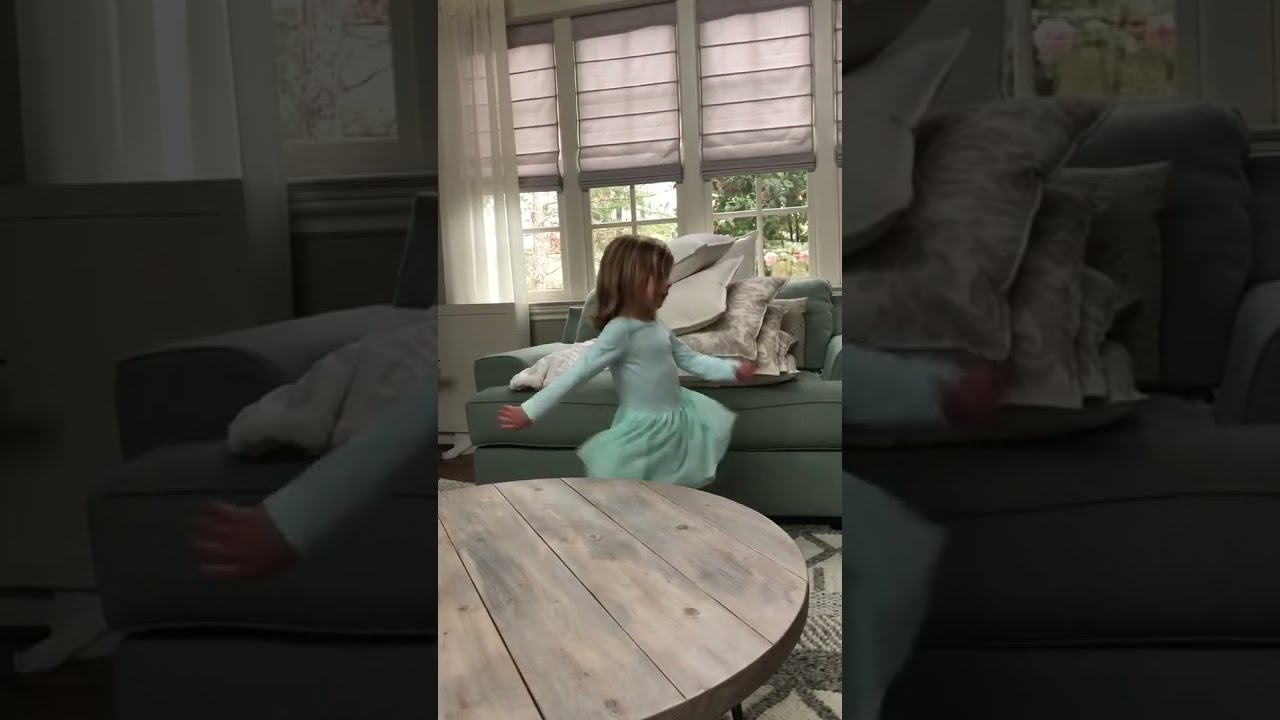This image is split into three sections with the right and left sides completely black, focusing attention on the middle section that depicts a cozy living room scene. Central to the image is a little girl with long, dirty blonde hair, dressed in a sheer, light greenish dress with long sleeves, reminiscent of a ballerina's attire. Her arms are outstretched, one in front and one behind, suggesting she is in motion, possibly swirling or dancing. She stands between a round, rustic-looking wooden table in the forefront and a sage-green chair, or sofa, behind her, which is stacked with pillows. Behind the girl, a window fills the background, its white shades pulled halfway up, revealing trees outside. Additional details include see-through curtains adorning the left side of the window and a rug underfoot, completing the serene and animated tableau.